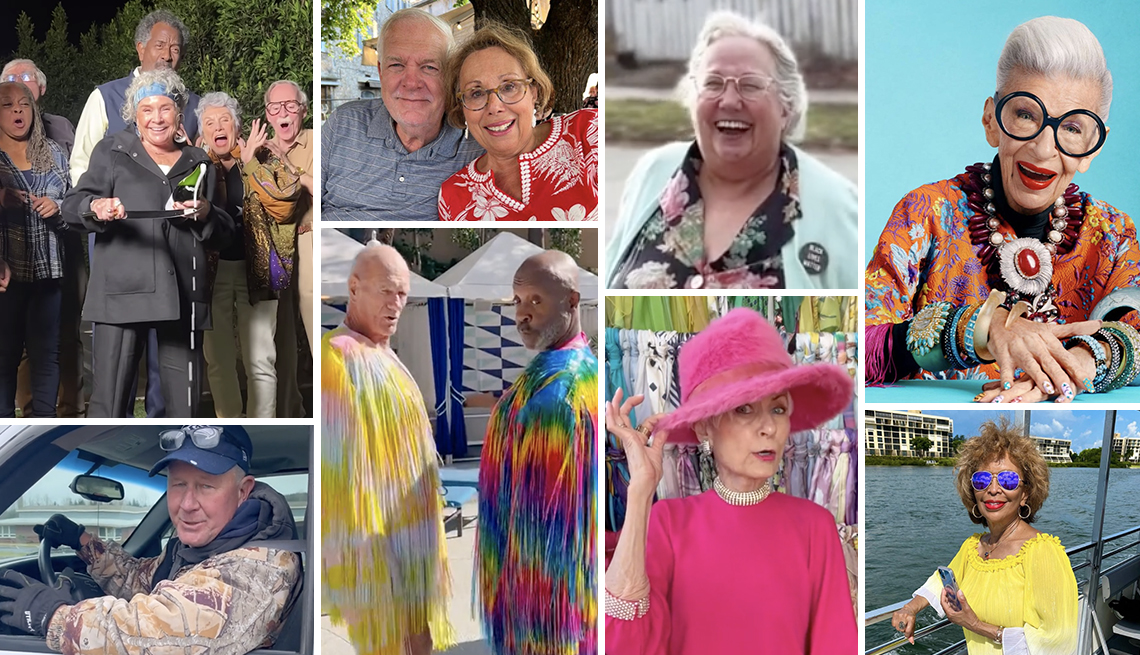This collage of eight photographs captures joyous and vibrant moments of elderly individuals in various lively and colorful settings. In the top left image, a group of three women and three men, including a very tall man standing behind a shorter woman with a cane and iPad, are basking in the sunlight with abundant shrubbery in the background. They all appear very happy, with some laughing and others smiling ecstatically.

Adjacent to this, an elderly couple beams at the camera, with the man in a blue striped polo shirt and the woman in a red and white tunic top, glasses, and sandy brown hair, suggesting a loving relationship. Below this, another image shows two bald men in eye-catching tie-dye shirts, standing side by side with heads turned sideways, with a white tent in the background, reflecting their playful spirits. 

On the right-hand bottom, a joyful elderly man is captured driving a truck, sunglasses perched on his head and wearing black driving gloves. Next to him, an elderly woman with large black glasses, red lips, and a colorful outfit showcases her exuberance, her mouth open in mid-laughter. Beneath her, a black woman with brownish hair and blue sunglasses is seen near water, possibly on a boat, holding a cell phone, and dressed in a lively yellow top. 

A photograph of a white woman in a pink fuzzy hat, matching pink top, and pearls adds to the charm with her playful pose, touching her hat as if in jest. Above her, another white woman with gray, short thin hair, wearing full-face glasses and a black floral top with a light blue sweater, smiles widely, her joyous spirit evident.

This vibrant and detailed series of photographs beautifully showcases the joy, humor, and colorful lives of elderly individuals.